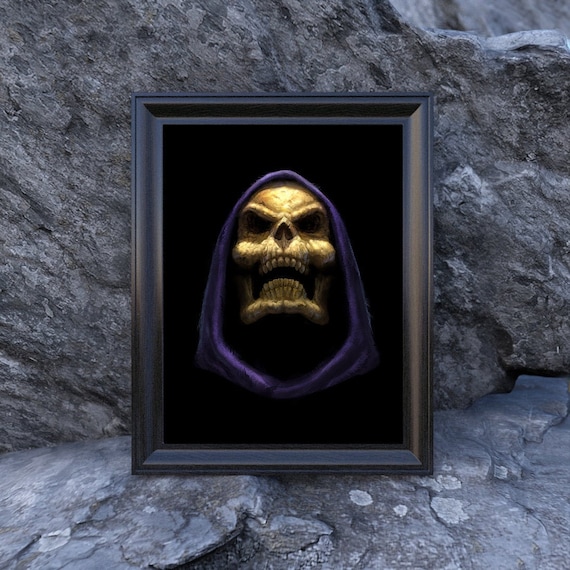This square image features a black wooden picture frame leaning on a flat, light gray rock, which serves as the base. The frame is set against a taller, grayish-brown stone in the background. Inside the frame is a vertical rectangular picture of a creepy-looking skull with an overall solid black background. The skull itself is a mix of brown, yellow, and white hues, with hollow black eye sockets, an open mouth with black gaps between the teeth, and a nose pointed slightly upward, featuring dark nostrils. The skull is adorned with a dark purple, hooded cowl reminiscent of Skeletor from the He-Man series. Both the neck and any additional body parts are obscured by the solid black backdrop within the frame. The detailed, eerie presentation of the skull, with its flaring nostrils and open mouth, creates an unsettling focal point in this artistic composition.